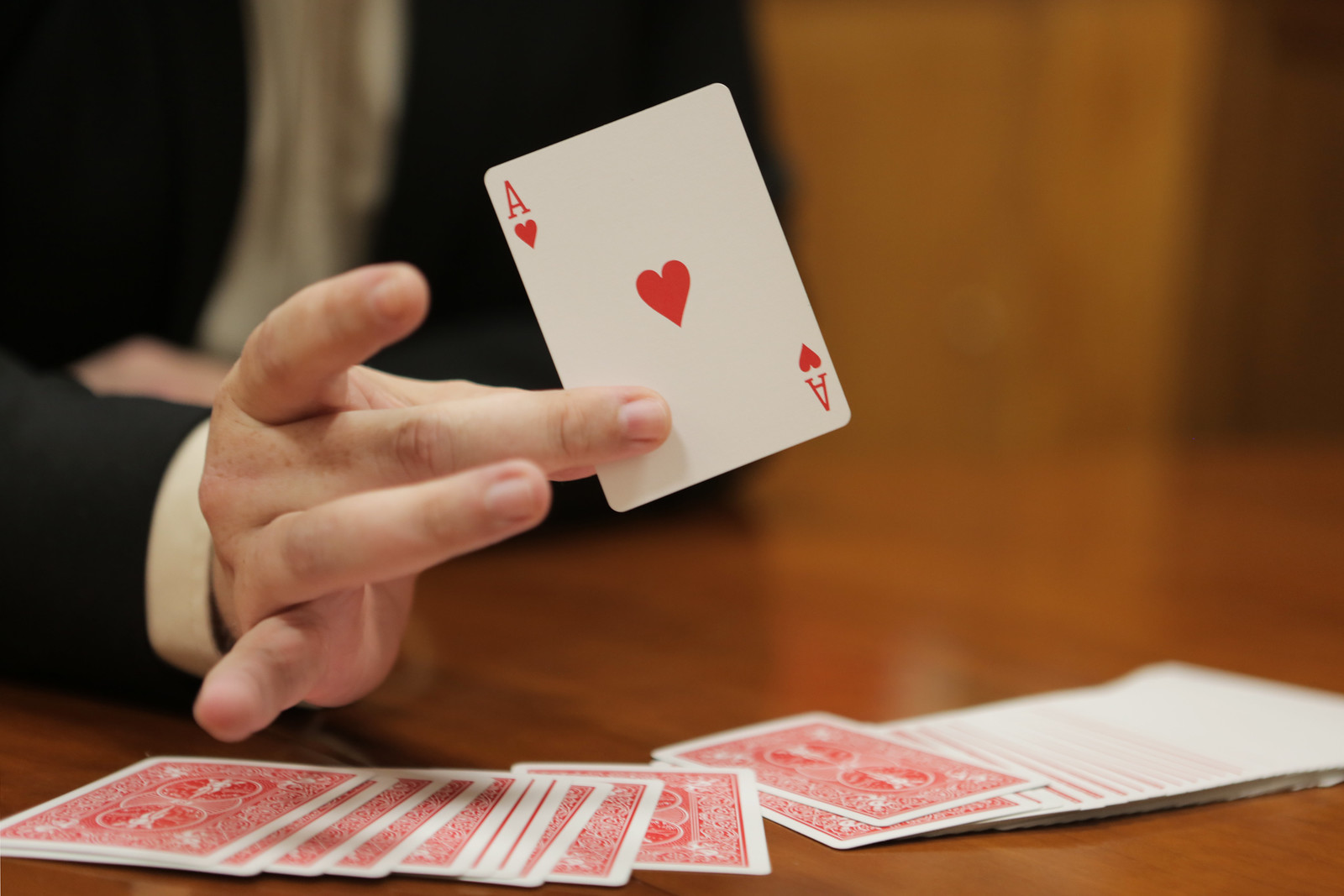A fan of standard playing cards is artfully spread across a wooden table, each card showcasing its vibrant red back design. A man, dressed in a black suit with a white button-up shirt underneath, steps partially into focus. His face remains blurred, drawing attention to his hand, which holds the Ace of Hearts delicately between his thumb and middle finger. The card is tilted slightly, roughly 20 degrees, adding a dynamic touch to the scene. The spread of cards on the table seems almost divisible into two distinct piles, with about ten cards in each pile clearly displaying the patterned backs.